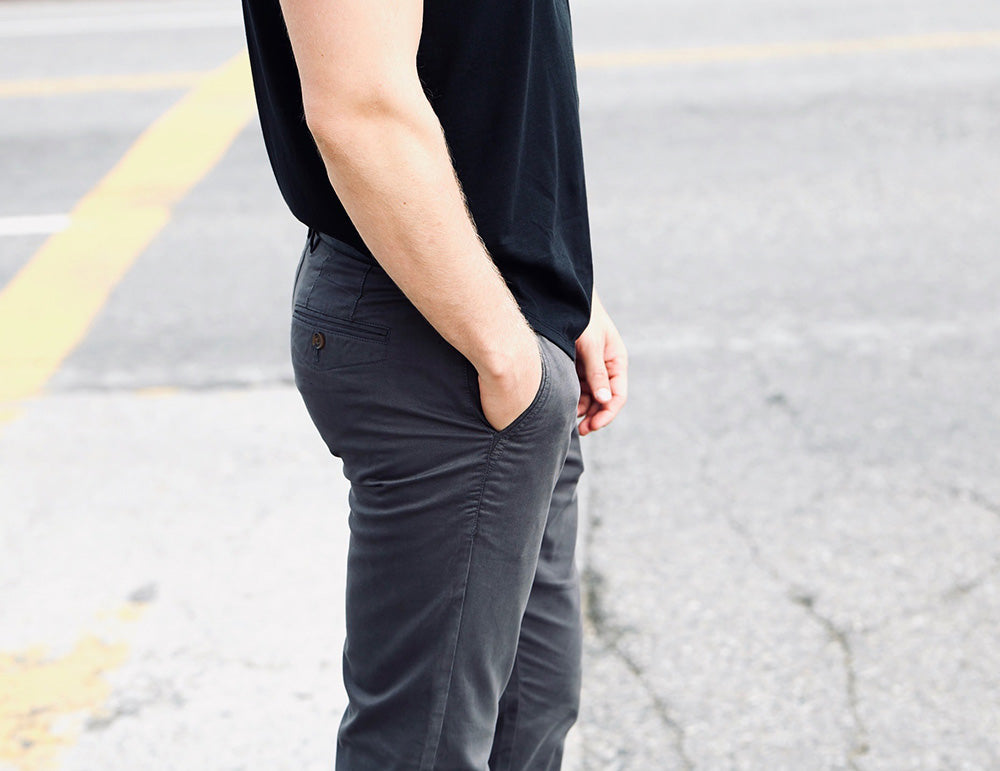The image depicts a Caucasian man standing on a cracked concrete road with a yellow lane marking in the background, possibly at an intersection. The scene is brightly lit, suggesting it's a sunny day. The man's attire includes a black t-shirt and dark gray, tight-fitting pants that appear somewhat low on his waist, emphasizing a "bumps" appearance. His right hand is inserted into his front pocket while his left arm hangs at his side. The man's hairy right arm and the smoothness of the image lend it a slightly surreal, almost AI-generated quality, enhanced by the shallow depth of field that blurs the background while keeping the subject in sharp focus.